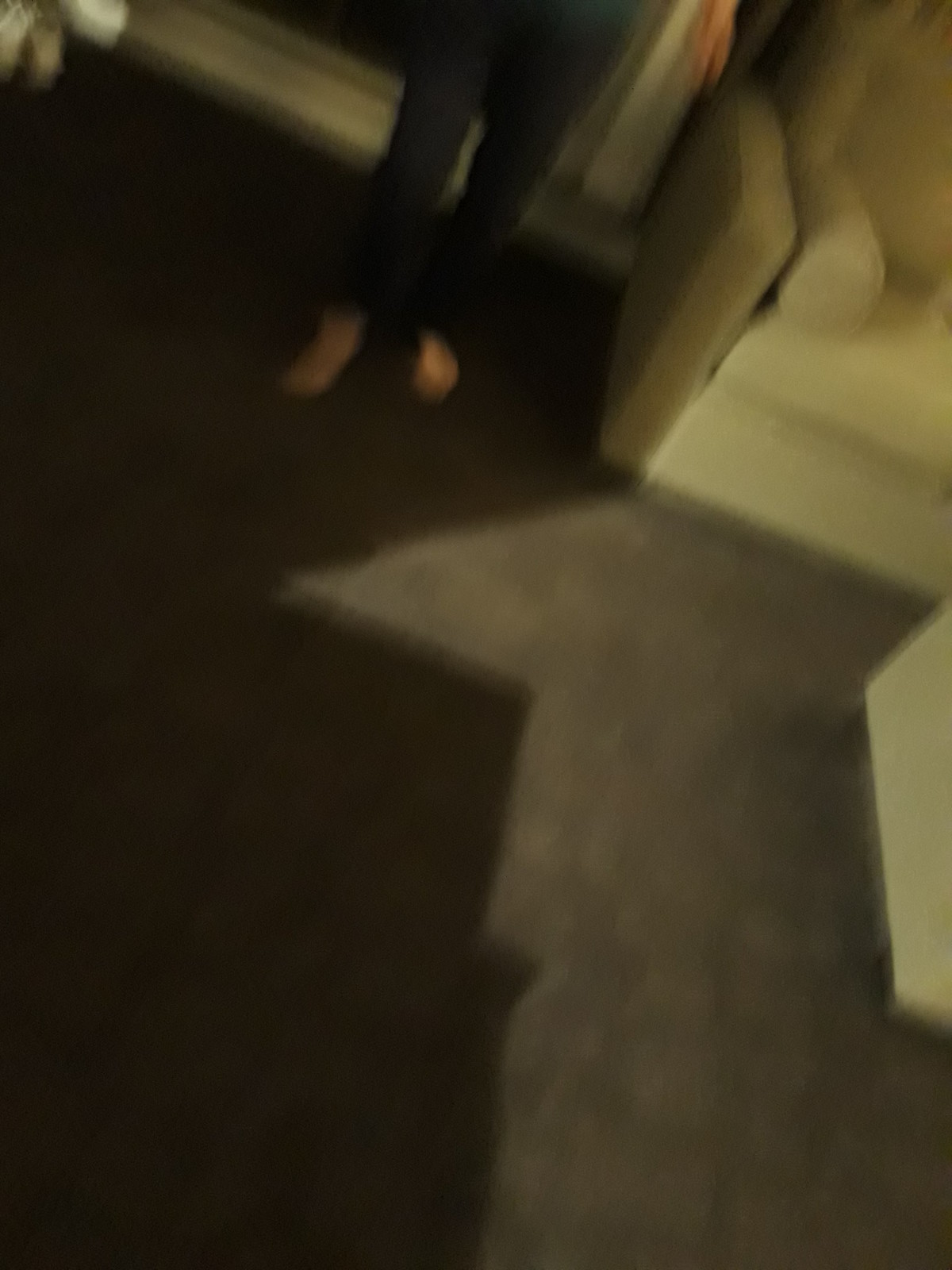In this extremely blurry image of a living room, a woman is partially visible from her upper thighs down, wearing tight black pants and either sandals or bare feet, revealing white skin. She stands on a textured dark brown or chocolate-colored carpet that has white markings, possibly footprints. A significant shadow falls across the carpet to the left, indicating a light source. An upholstered tan armchair is situated to her right, partially visible in the upper right corner of the image. In front of the chair is a matching tan ottoman or table, viewable only from one side. Behind the woman appears to be a large window or door with molding at the bottom and sides, and a reflection is noticeable to her left.